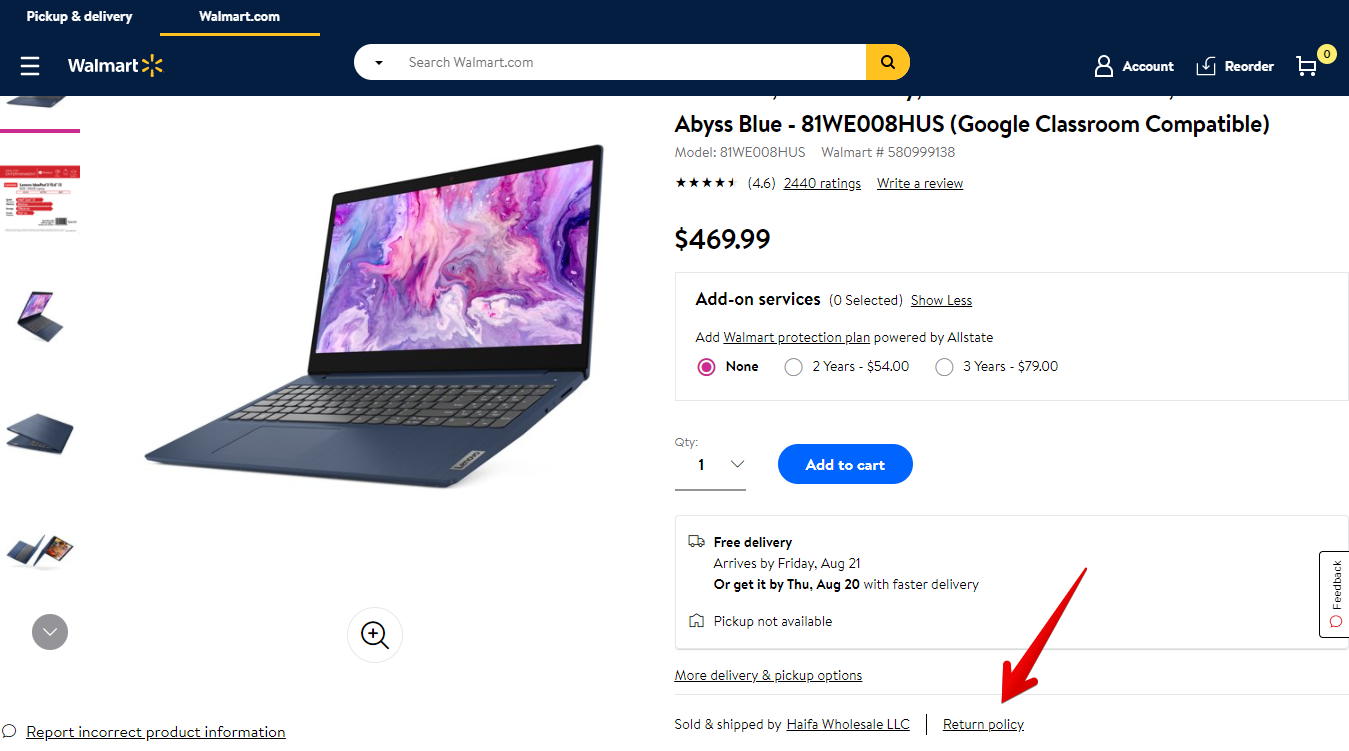A screenshot of Walmart's website featuring an Abyss Blue-colored laptop model 81WE008HUS, which is compatible with Google Classroom. At the top of the website page, a blue header includes a search bar with the placeholder text "Search Walmart.com." On the upper left-hand side, there are two selectable tabs labeled "Pickup & Delivery" and "Walmart.com." Beneath the "Pickup & Delivery" tab, the Walmart logo is displayed in white with the star symbol. The showcased laptop, priced at $469.99, has a red arrow pointing towards the "Return Policy" link, located at the bottom center of the image.